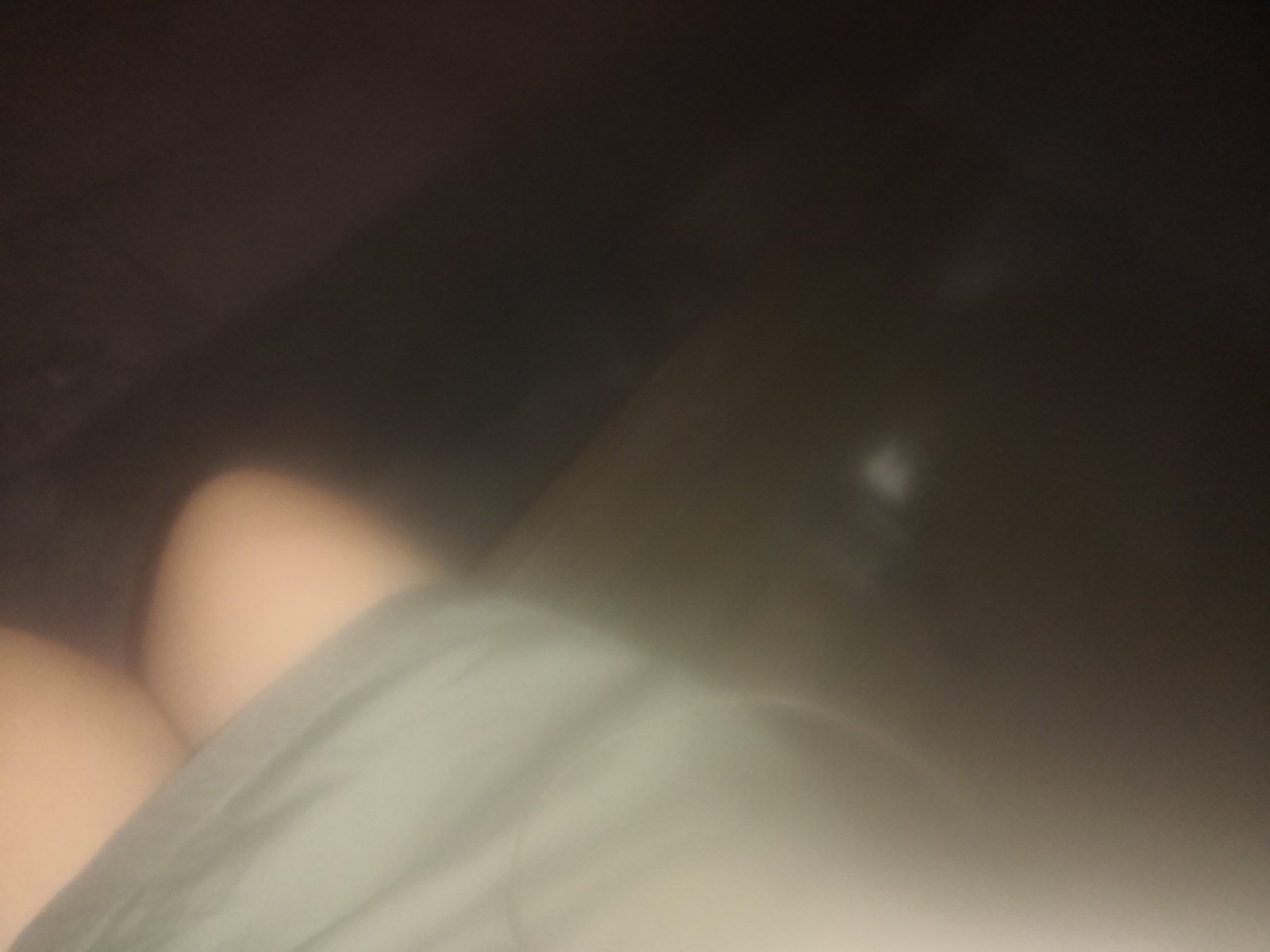This photograph is extremely blurry and out of focus, suggesting it might have been taken accidentally or with a camera in motion. The image is dark, possibly taken at night or in a poorly lit room, with a flash or an alternate light source illuminating part of the scene. The top half of the image is entirely black. In the bottom half, diagonally from the bottom right to nearly the left corner, we can see a woman's right leg and part of her left leg, with her knees together. She has pale skin and is wearing a light gray or olive green dress that hits just above the knees, possibly made of satin with a gauzy overlay. Only the right leg and part of the left knee are visible. The woman appears to be sitting on a dark gray bench, with the flooring, which is darker than the bench, slightly visible on the left side of the image. A small white speck is noticeable on the bench. Overall, the obscured, angled, and poorly lit nature of the photograph makes it difficult to discern further details.